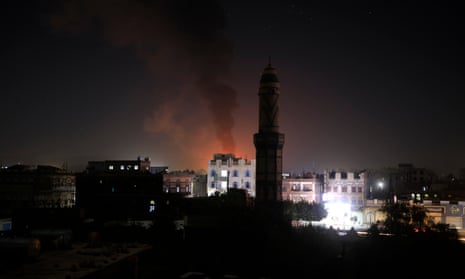In this dark nighttime scene, the foreground is completely silhouetted, making it difficult to distinguish any shapes, though some trees and a tall, cylindrical tower are faintly visible. The tower seems to be a notable structure, potentially a religious building or memorial, silhouetted against the night sky which is particularly dark around the edges of the image. 

In the midground, a bright light illuminates a cluster of rectangular, multi-story buildings, which have several windows—some of them lit. One central building stands out due to the amber light and dark smoke billowing from it, suggesting a fire or explosion. This red smoke is visible against the grayish sky in the background. The buildings, lacking the height of skyscrapers, give the impression of a landscape possibly situated in a region like the Middle East or Ukraine. Overall, the scene appears chaotic, possibly the aftermath of a bombing or similar incident, inferred from the large amount of smoke and the intense lighting emanating from the central structure.